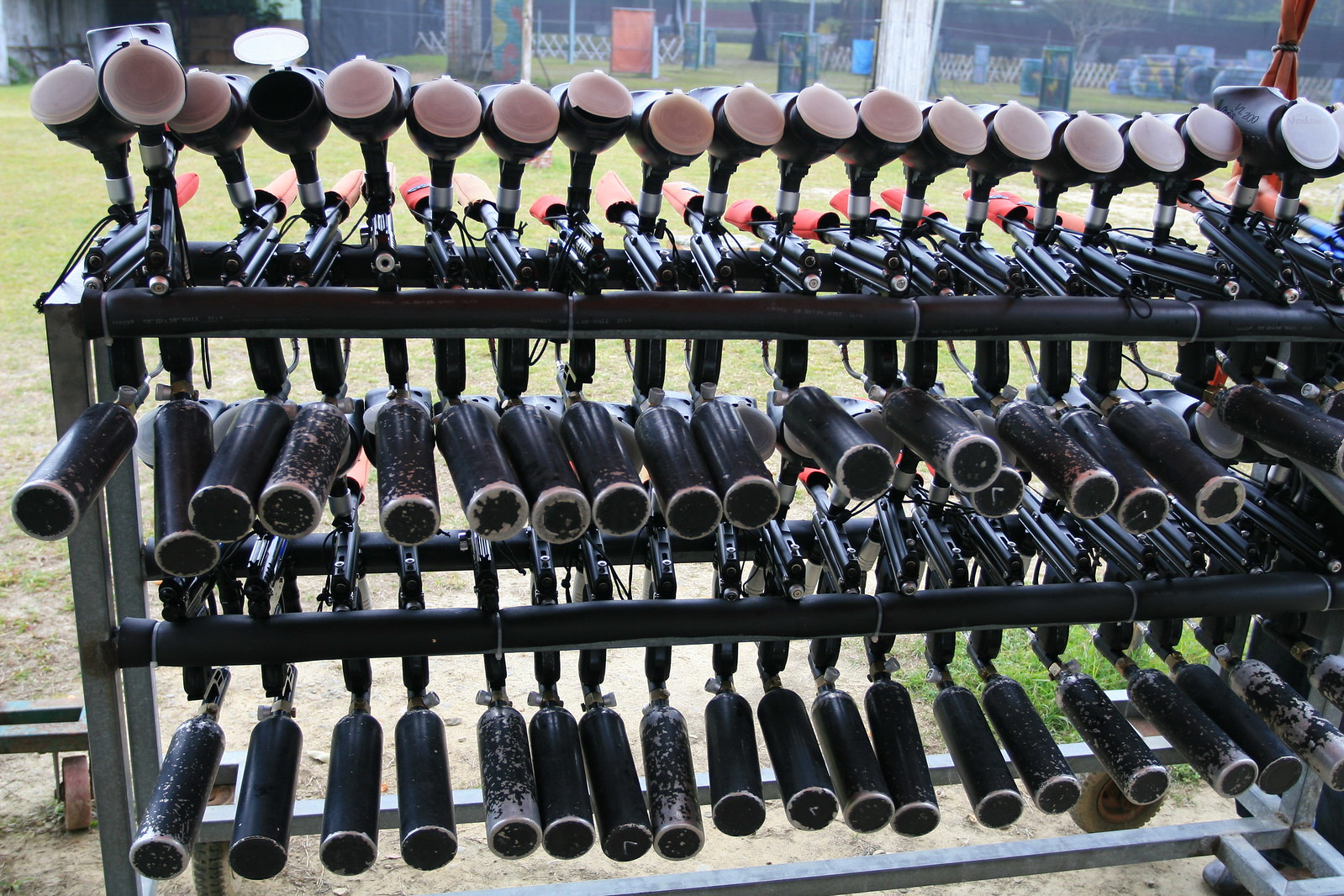This image depicts a metal shelving unit situated outdoors in a grass-covered field, likely part of a shooting range or paintball facility. The shelving unit features three rows of cylindrical items. The bottom two rows are filled with black canisters, presumably paintball gun cartridges. The top row contains additional components, possibly paintball hoppers with black plastic bodies and clear lids. These items collectively have a black color with occasional pink and red accents. In the background, there is a lawn extending out into the distance with various rectangular targets set up for shooting practice. A white crisscross picket fence is visible further back, marking the edge of the field. The green grass appears patchy, suggesting inconsistent watering.